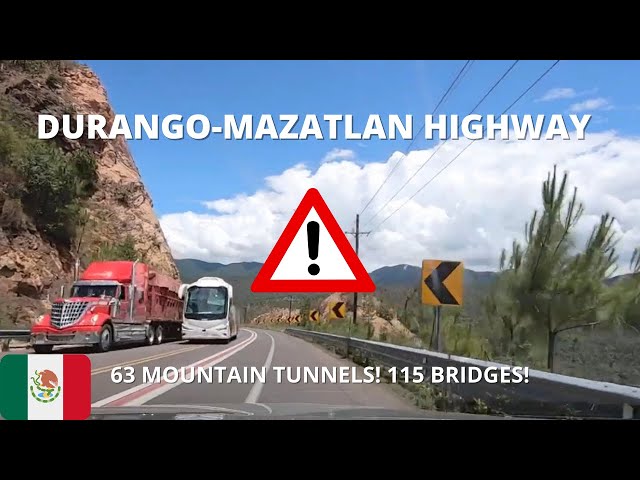The image depicts a hazardous scene on the Durango-Mazatlan Highway, an outdoor setting with a blue sky and clouds above. Dominating the frame is a winding road carved along the side of a mountain. The road is narrow and flanked by silver guardrails, with a perilous hundred-foot drop-off on one side. The mountainside is brown with patches of green trees. To the left, the mountain slopes steeply upward, while on the right, green trees with brown branches add to the landscape's rugged beauty.

A large red semi-truck with silver trim and a white, black-tinted tour bus are dangerously close as they navigate a curve in a no-passing zone. The bus appears to be attempting to overtake the semi, creating a tense, high-risk situation. The scene is captured from another vehicle heading towards them, emphasizing the imminent danger.

Signs on the right side of the road, including bright yellow caution signs and a notable red and white triangle with a black exclamation point, underscore the danger. There is also a prominent Mexican flag with green, white, and red stripes and an emblem in the middle.

Above the image, white text reads "Durango-Mazatlan Highway." Beneath it is another warning: "63 mountain tunnels, 115 bridges." Additionally, multiple road markings can be seen, including white and yellow lines, and a red line, adding to the driving complexity.

The vivid details and numerous warnings starkly highlight the hazardous nature of this treacherous mountain road.